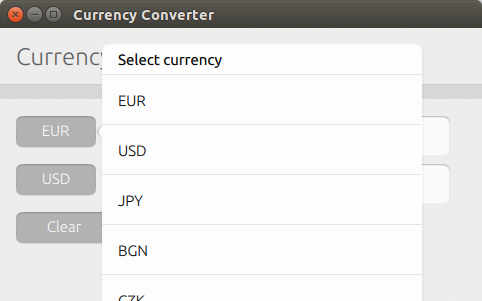This image is a detailed screenshot of a currency converter feature on a website, designed to facilitate the conversion of various international currencies. At the very top of the screenshot, a long rectangular black bar is prominently displayed. Positioned on the right side of this bar are three distinctive circles: the first circle is red with a black 'X' symbol, the second is a darker gray featuring a line, and the third circle, also a darker gray, showcases a square.

In white text, the bar is labeled "Currency Converter," indicating the purpose of the page. Directly below this, the word "Currency" is visible, partially obscured by an opened drop-down menu. This drop-down menu, labeled "Select Currency," provides several currency options. The first displayed option is "EUR," followed by "USD," "JPY," "BGN," and a partially visible "CZK," all written in black text.

In the background, three darker gray rectangular boxes are visible, each denoting a different currency type. The first box is labeled "EUR," the second is "USD," and the third option appears to be a clear, or unselected, box. This detailed setup conveys the interface and available options for users interacting with the currency converter tool on the website.